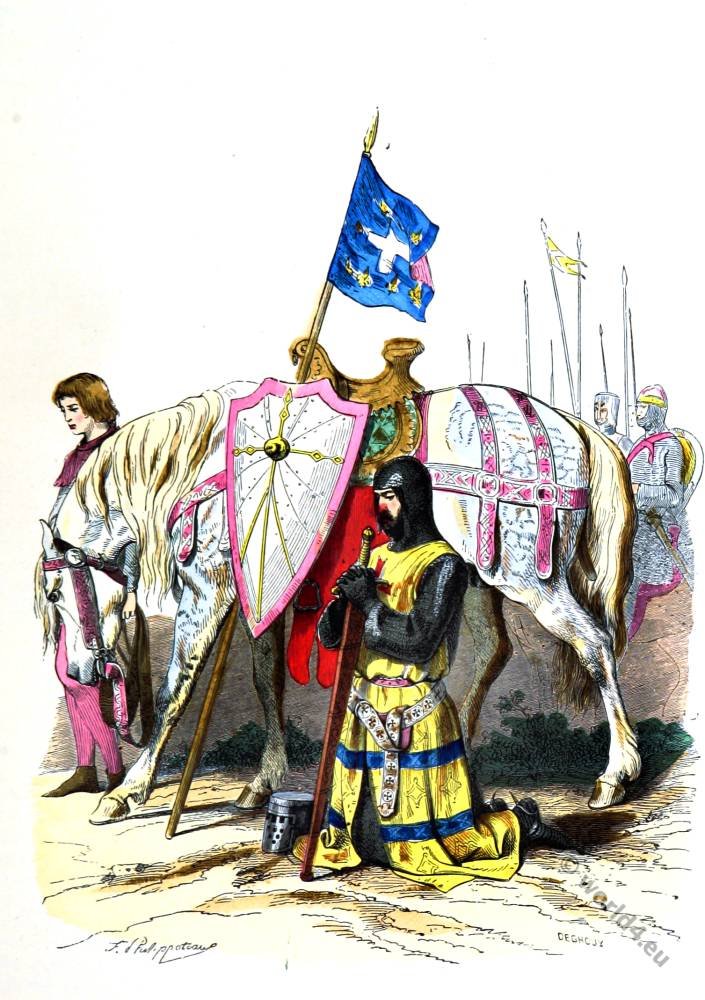The artwork is a detailed colored sketch or pencil drawing set in a medieval scene. The main subject is a knight, reminiscent of a crusader, dressed in layered black chain mail with a yellow robe draped over it. He is kneeling on both knees, holding a sword close to his chest as if in prayer or contemplation, with his silver helmet placed on the ground beside him to his right. Behind the knight stands his horse, adorned with pink saddles, a shield with a pink outline, a yellow cross on a white background, and a blue flag with a white cross and gold stars. To the left of the image is a young individual with short brown hair, wearing pink pants, looking off to the left. Additionally, in the background, there are other soldiers seen standing at attention or marching, equipped with spears and featuring pink accessories as well. The overall composition and elements suggest an elaborate medieval setting full of symbolic details.